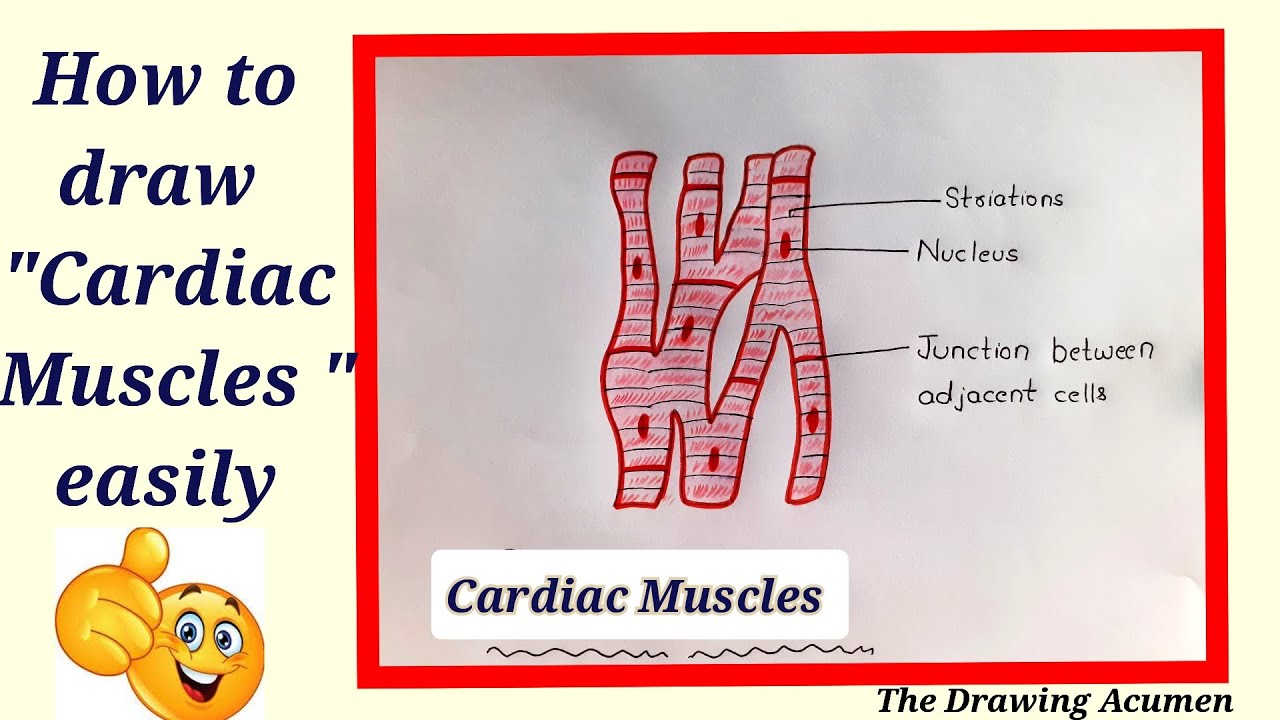This image is a detailed guide on how to draw cardiac muscles easily. The left side of the image features large text reading "How to Draw Cardiac Muscles Easily," accompanied by a cheerful yellow smiley face giving a thumbs-up. The right side showcases a meticulously hand-drawn illustration of cardiac muscles, bordered with a red frame. The drawing includes various annotations with arrows pointing to specific parts of the muscle labeled as "striations," "nucleus," and "junction between adjacent cells." The cardiac muscles are depicted using red and black colors, with red outlining and pinkish interior details. The drawing is labeled "Cardiac Muscles" at the bottom, and the phrase "the drawing acumen" is noted in the bottom right corner. The background is an off-white or pale ivory shade, adding a clean and educational feel to the presentation, reminiscent of a textbook or a PowerPoint slide.